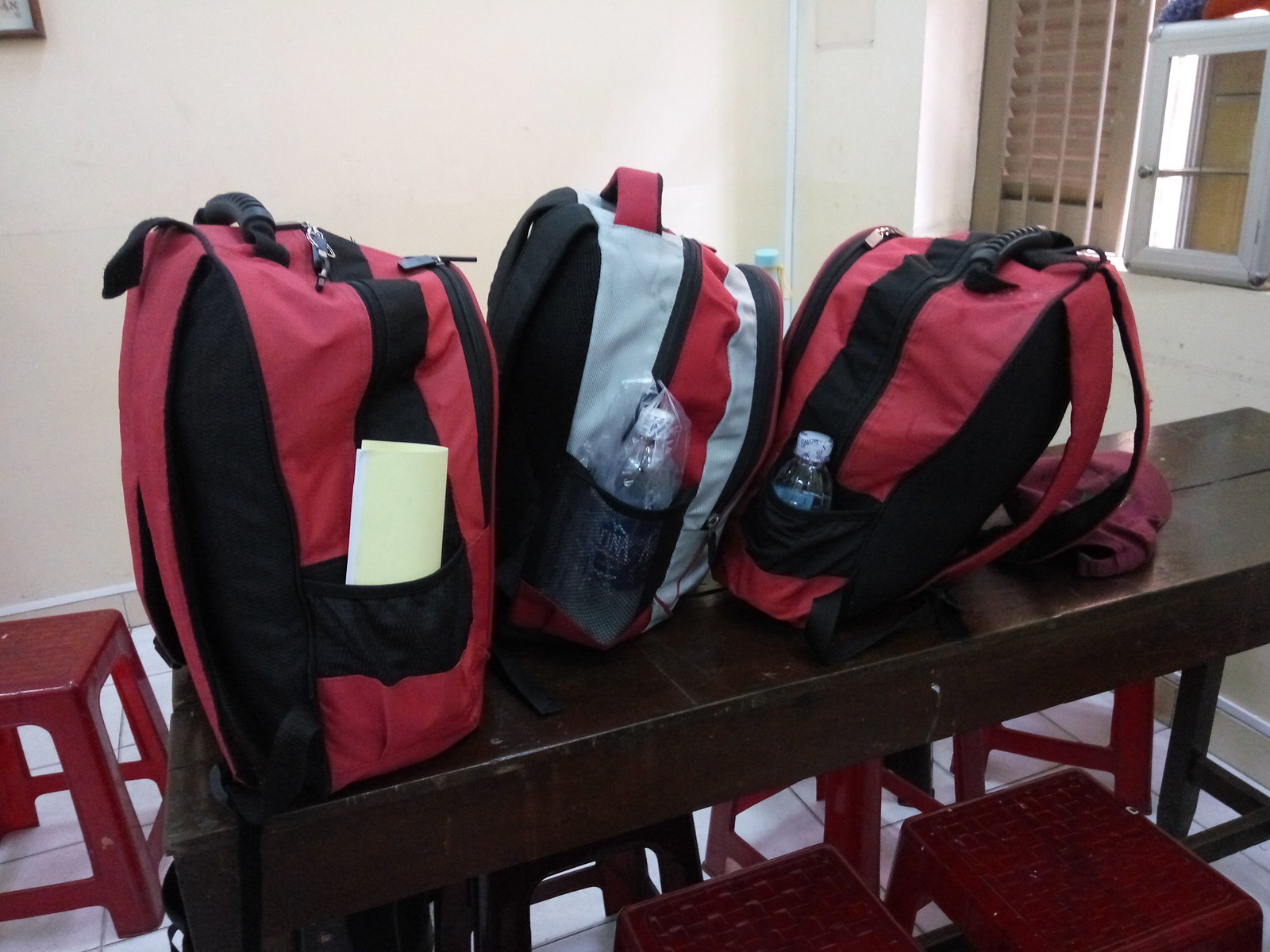This is a photograph of three backpacks lined up next to each other on a narrow, tall, dark walnut wooden table with dimensions likely around 4-5 feet in length and about 18 inches in width. The table is surrounded by several small red stools, possibly maroon, which appear to be closer to chair height rather than full-height stools, enhancing the table’s high impression. 

From left to right, the first and third backpacks are identical with a red body and black stripes; the leftmost backpack contains a folded yellow slip of paper in its side pocket. The central backpack differs, having a gray base with red and black accents, and its side pocket holds a water bottle possibly inside a plastic bag. The rightmost red and black backpack also has a water bottle in its side pocket and seems to contain a good amount of contents, causing it to lean slightly as it lacks support from other items.

The setting is a plain room with white linoleum floors and cream or tan-colored walls, adding to a bland backdrop. A window is visible to the right side of the room, equipped with blinds, and there appears to be a white cabinet or storage unit nearby. The overall impression is one of simplicity and functionality, with no additional decorations present in the environment.